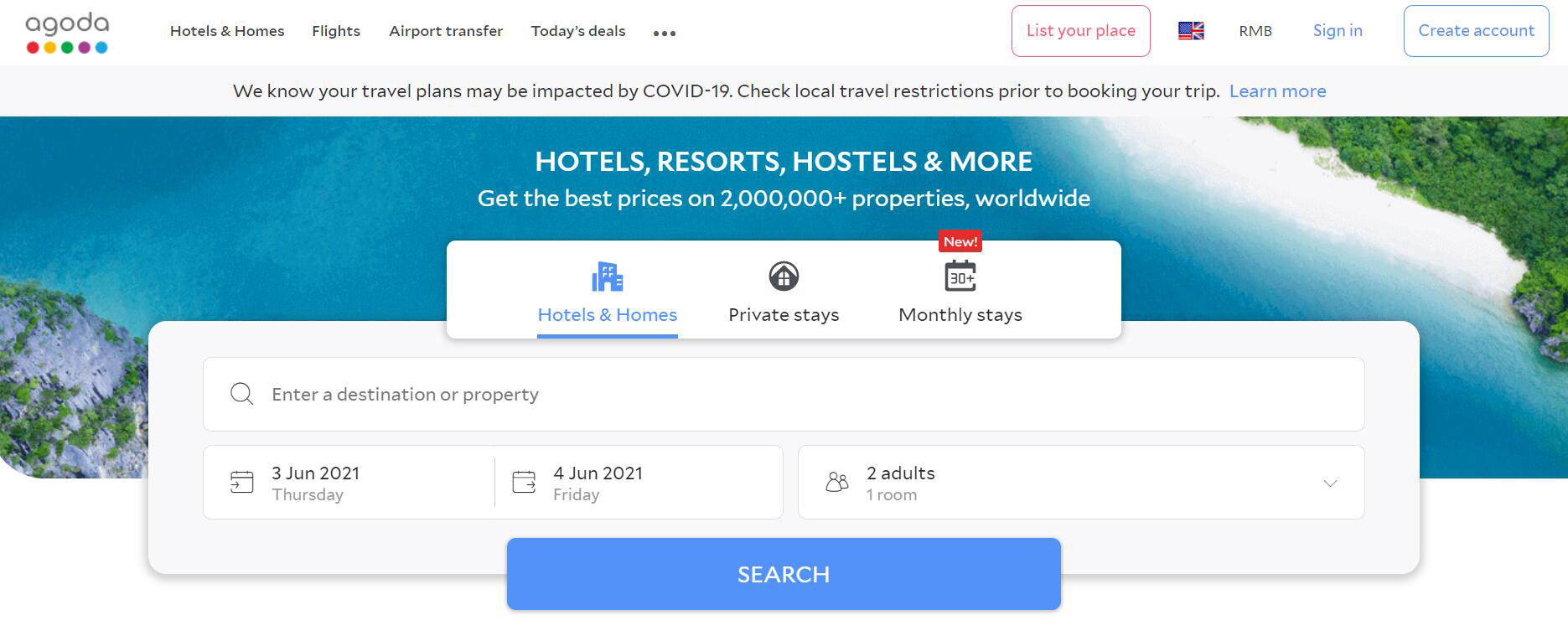**Descriptive Caption:**

This image is a screenshot from a travel website. At the top of the image, the header contains the following navigation and function options starting from the left: "Agoda" in large font, followed by "Hotels and Homes," "Flights," "Airport Transfer," and "Today's Deals." Further to the right, there is a white box outlined in red containing the text "List Your Place" in red lettering. Adjacent to this box is an icon of a flag, followed by the currency "RMB," and options to "Sign In" as well as an option within a blue box to "Create Your Account."

Beneath this header, there is a gray notification bar centrally displaying the message: "We know your travel plans may be impacted by COVID-19. Check local travel restrictions prior to booking your trip." To the right of this message is a clickable "Learn more" link in blue.

The primary image below this bar depicts a serene coastal scene. There is clear, blue water prominently featured, with a small section of beach visible in the upper right corner backed by lush green trees. On the lower left corner of the image, there is more land covered in green trees, possibly rocky or sandy in nature.

Below this scene, superimposed on the lower part of the image, is a white navigation bar with tabs labeled "Hotels and Homes," "Private Stays" with an icon of a house, and "Monthly Stays." Underneath this bar is another input section that reads "Enter a destination or property." It also shows date selections, "3 June 2021" and "4 June 2021," alongside the option specifying "Two adults, one room." The section concludes with a prominent blue "Search" button.